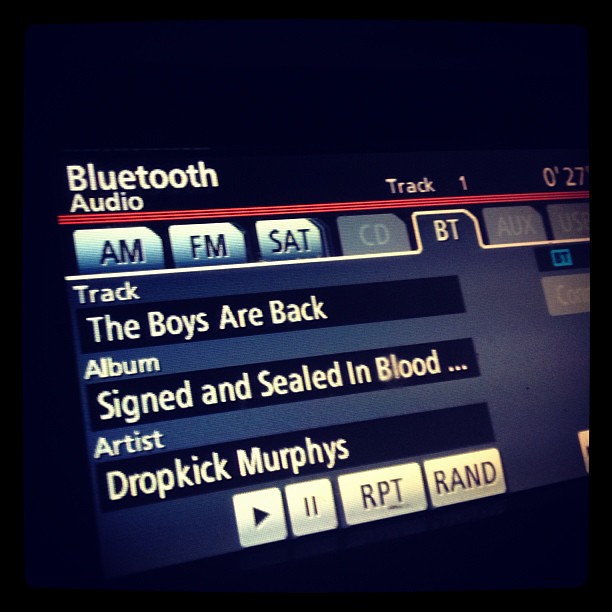The detailed photograph captures the digital LCD panel of a car's dashboard, illuminated in the dark. At the top left, the screen displays "Bluetooth audio" in white text. Directly to the right, it shows "Track 1" and further to the right, "0'27." Just below this, a striking red band is visible. Below the red band, there are seven graphical tabs for media options, with the first three tabs featuring a gradient from white to dark blue, labeled "AM," "FM," and "SAT" in black text, respectively. The fourth tab is gray and labeled "CD," while the fifth tab, highlighted in solid dark blue with a white border, indicates the selected "BT" (Bluetooth) option. The "AUX" and "USB" tabs, both gray, follow next.

Beneath these tabs, on the left side of the screen, "Track" appears in white text above a long horizontal black rectangle displaying "The Boys Are Back" in white. Below, the word "Album" appears, paired with another black rectangle containing "Signed and Sealed in Blood..." in white text. Further down is the word "Artist," with the final black rectangle showing "Dropkick Murphys" in white. To the right of this text block, there are four control buttons with a white and gray gradient: a triangle (play), two vertical lines (pause), "RPT" (repeat), and "RAND" (random). The overall color scheme includes a mix of black, white, dark blue, and red, with the blue screen setting the media display scene in a sleek, modern car interface.